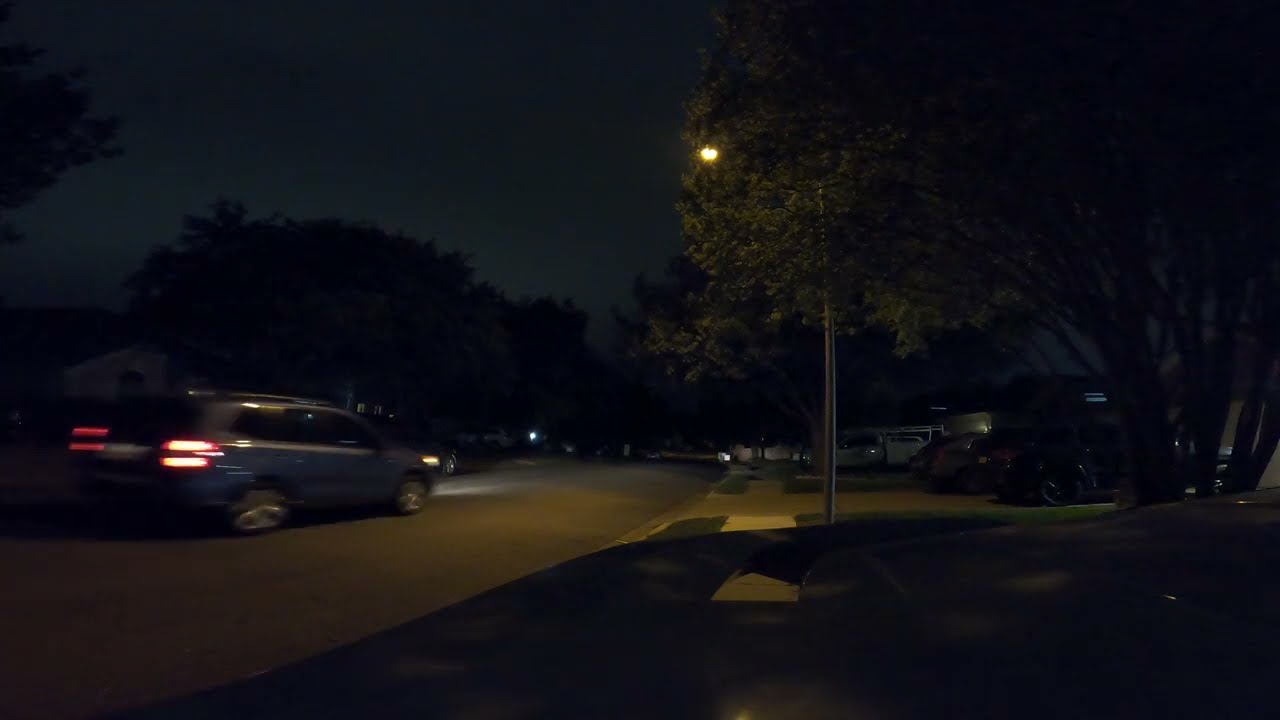This horizontally aligned rectangular nighttime photograph captures a dimly lit residential street scene. The dark sky dominates the top left corner, contrasting with large, leafy trees on the top right. A tall lamppost in the middle emits a soft yellow light that filters through the branches, partially illuminating the area.

On the left side of the image, a blurry blue or gray station wagon, possibly an SUV, drives down the residential street with its taillights glowing red. The presence of a T-shaped driveway on the right breaks through the sidewalk and is faintly lit by the streetlight rather than headlights.

In the lower right and extending across the middle, a dark object, likely the hood of a car, suggests the photo was taken from inside a vehicle. Numerous parked cars line the right side, including a white truck backed into a driveway. Although it’s too dark to discern whether this area is a business or a residential parking lot, the overall scene is characterized by the indistinct shapes of vehicles against the backdrop of shadowy trees and a dimly lit street.